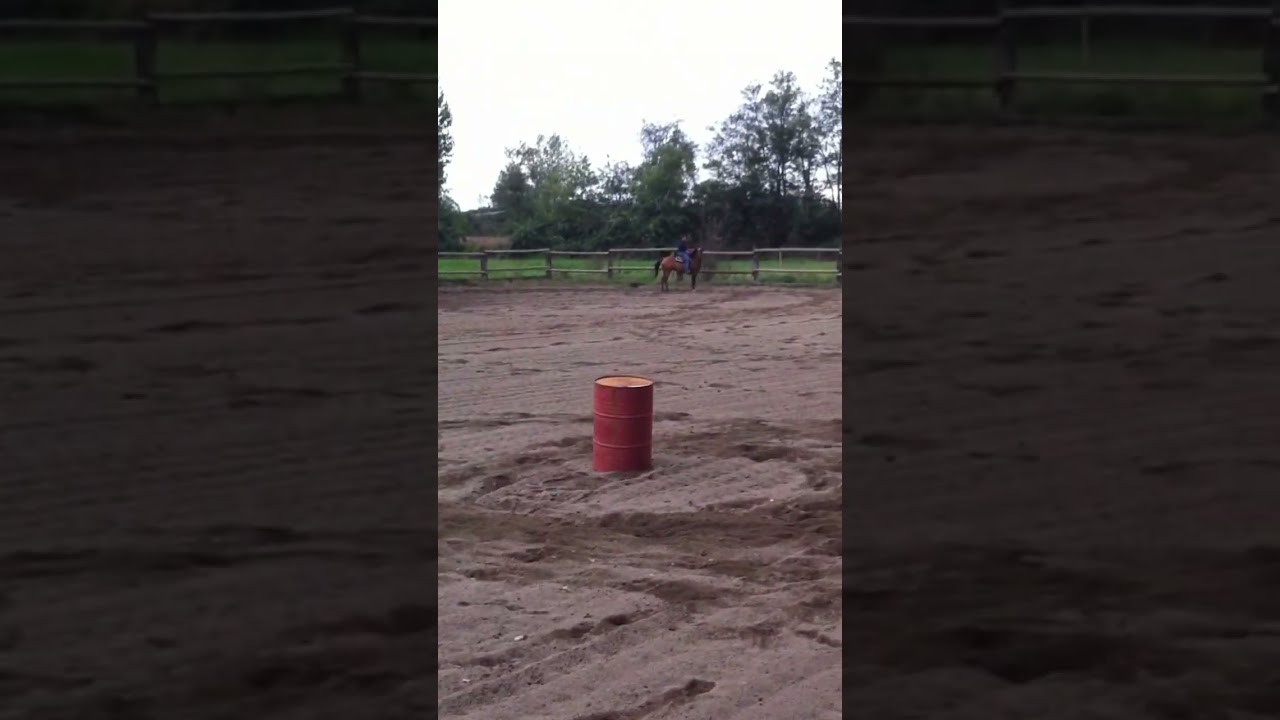The image captures an outdoor horse ring or stadium taken in portrait mode. In the center of a sandy gravel circular arena, there is a prominent red oil drum cylinder surrounded by a mix of dry, patterned sand, tire marks, and footprints, with areas of wet sand near the barrel. At the far edge of the arena lies a wooden fence with two horizontal bars between the posts. Behind the fence, a brown horse stands still, ridden by a person wearing blue. Beyond the fence, a grassy field transitions into a woodland area featuring trees and bushes, all beneath a bright, overcast white sky. The main vertical third of the image presents a zoomed-out view, while the left and right thirds include magnified sections, highlighting the ground details.